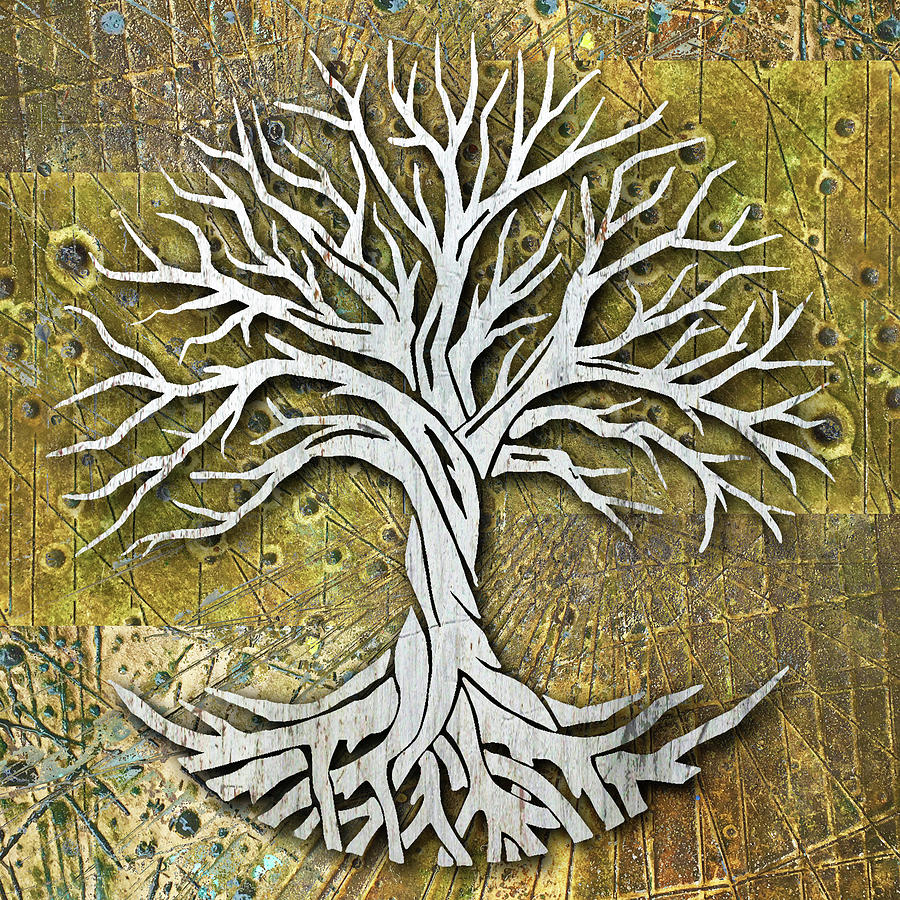The image displays a highly detailed and intricate interpretation of the Yogg-Dreschel Celtic Tree of Life. The centerpiece of the artwork is a gracefully twisted tree, featuring an elaborate network of branches and roots that spiral and weave around the trunk. This tree, seemingly carved from naturally unfinished wood, is devoid of leaves, emphasizing its intricate limbs and flowing roots. The tree is symmetrically arranged in such a way that it forms an almost perfect circle.

This central motif is set against a richly textured background, designed to resemble weathered wood. The background is composed of varying shades of brown, arranged in a patchwork of square segments, each showcasing unique wood grains, lines, and imperfections, adding depth and character to the piece. This interplay of textures makes the background look like it has been pounded and etched with lines and circles, enhancing the visual complexity.

The entire artwork is mounted on a square-shaped brass metal base, further adding to the rustic and timeless appeal of the piece. The brass, while not overly shiny, complements the natural wood, creating a cohesive visual narrative that effortlessly blends organic and metallic elements. The background pattern, reminiscent of peacock's feathers, provides a dynamic contrast to the tree's otherwise static form, enriching the overall composition and drawing the viewer’s attention to the intricate details of the Celtic Tree of Life.